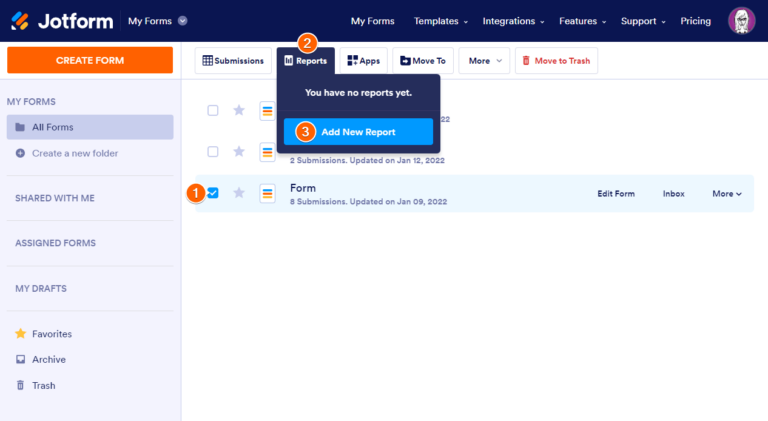The image features a user interface with a dark blue header at the top. On the left side of the header, there are blue, red, and orange diagonal lines. Bold white text on the header reads "Drop Form," with smaller text underneath that states "My Forms." Toward the right side of the header, there are menu items labeled "My Forms," "Templates," "Integrations," "Features," and "Support"—all accompanied by dropdown menus. Additionally, there's a "Pricing" option and a purple circle with a white icon of a woman, indicating a profile picture.

Below the header, on the left side of the screen, there's an orange rectangle with the text "Create Form." Directly opposite, on the right, there are three different form options. The bottom form is marked with a checkmark inside an orange circle containing the number one. At the top, under a section labeled "Reports," an orange circle with the number two informs the user that there are currently no reports yet. A light blue rectangle labeled "Add New Report" is accompanied by an orange circle with the number three inside it.